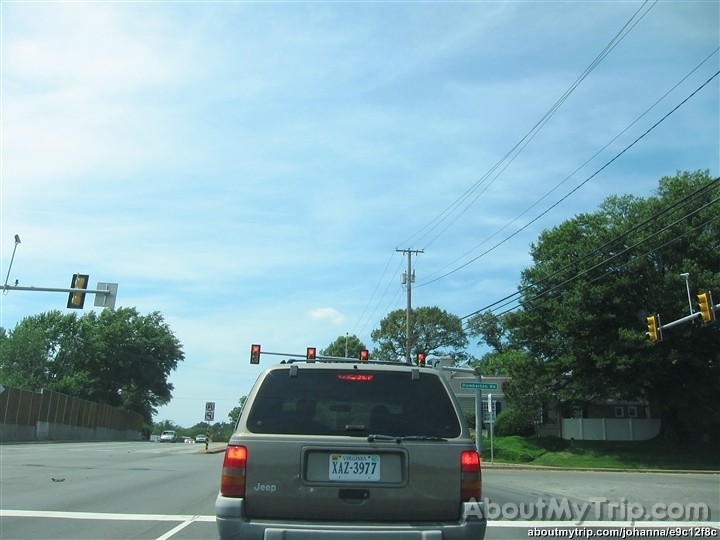The photograph, taken from a dash camera on a sunny day with some wispy clouds and white fluffy ones in the upper left corner, captures a detailed road scene. At a stoplight, a metallic gray Jeep with the license plate XAZ 3977 from Virginia is in front of the viewer's car, its taillights illuminated. The Jeep waits at an intersection where overhead traffic signals display red lights for all directions. To the upper right and center-right of the image, electrical poles and power lines are visible. The roadway, lined with tall, dark green trees on both sides, has two lanes in each direction, with vehicles traveling in opposite lanes to the left. The bottom right of the image displays the text "aboutmytrip.com/aboutmytrip.com/johanna/e9c12f8c", indicating the source of the trip.